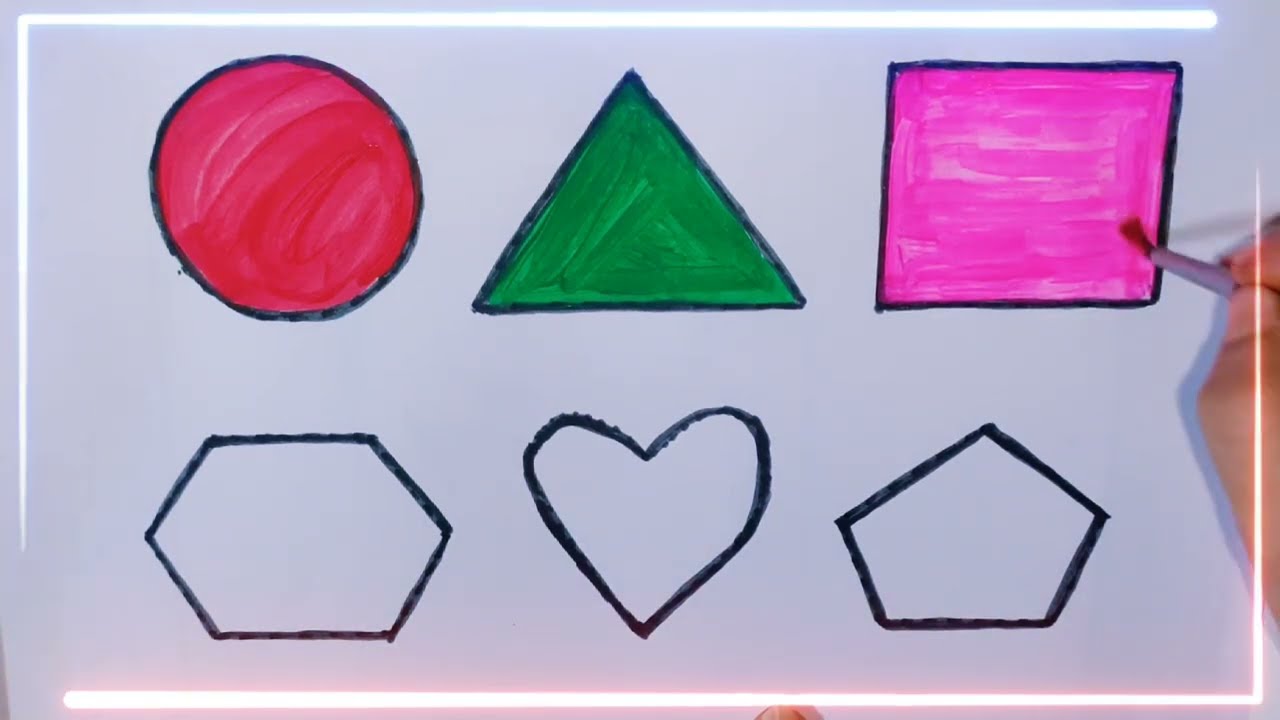The image depicts a collection of geometric shapes outlined in black paint, arranged in two rows against a white background. The top row features, from left to right, a red-painted circle, a green-painted triangle, and a partially painted magenta-pink square. A hand holding a paintbrush hovers over the square, continuing to apply the pink paint. The bottom row includes, from left to right, unpainted black outlines of a hexagon with six sides, a heart, and a pentagon with five sides. A subtle, glowing pink stripe borders the image along the right side, top, and bottom edges, enhancing the visual composition.